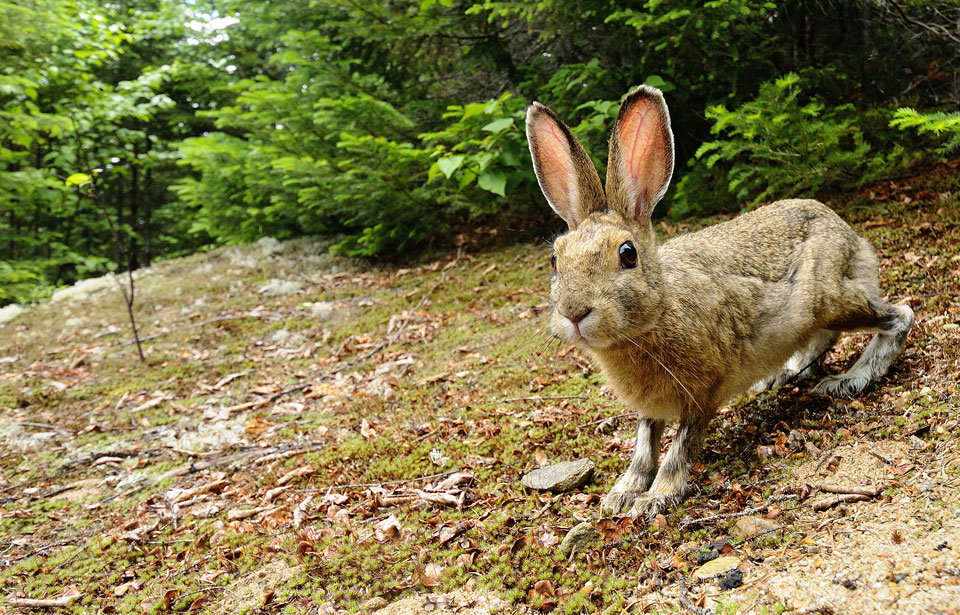This is a detailed digital photograph of a light brownish-gray rabbit, often referred to as a bunny, positioned on the right-hand side of the image. The rabbit has distinct large ears that stand tall, with pink inner ear linings, and expressive black eyes. While not overly plump, it appears alert and youthful, as suggested by its small size and delicate features including long whiskers, with one noticeable gray whisker stretching out from its nose.

The setting is an earthy, lightly sloping hill adorned with a mix of beige dirt, old leaves, twigs, and patches of yellowish grass. Surrounding the rabbit, the environment transitions into lush greenery with abundant plants, bushes, and trees in the background, creating a forest-like atmosphere. The overall greenery adds a vibrant backdrop of rich greens, contrasting against the softer colors of the ground.

The lighting suggests an overcast yet bright period, as indicated by the diffused shadow under the rabbit, hinting at midday without the harshness of direct sunlight. This naturalistic scene captures a peaceful and vivid snapshot of the rabbit’s habitat, devoid of any text or additional elements, emphasizing the serene and raw beauty of the rabbit in its environment.